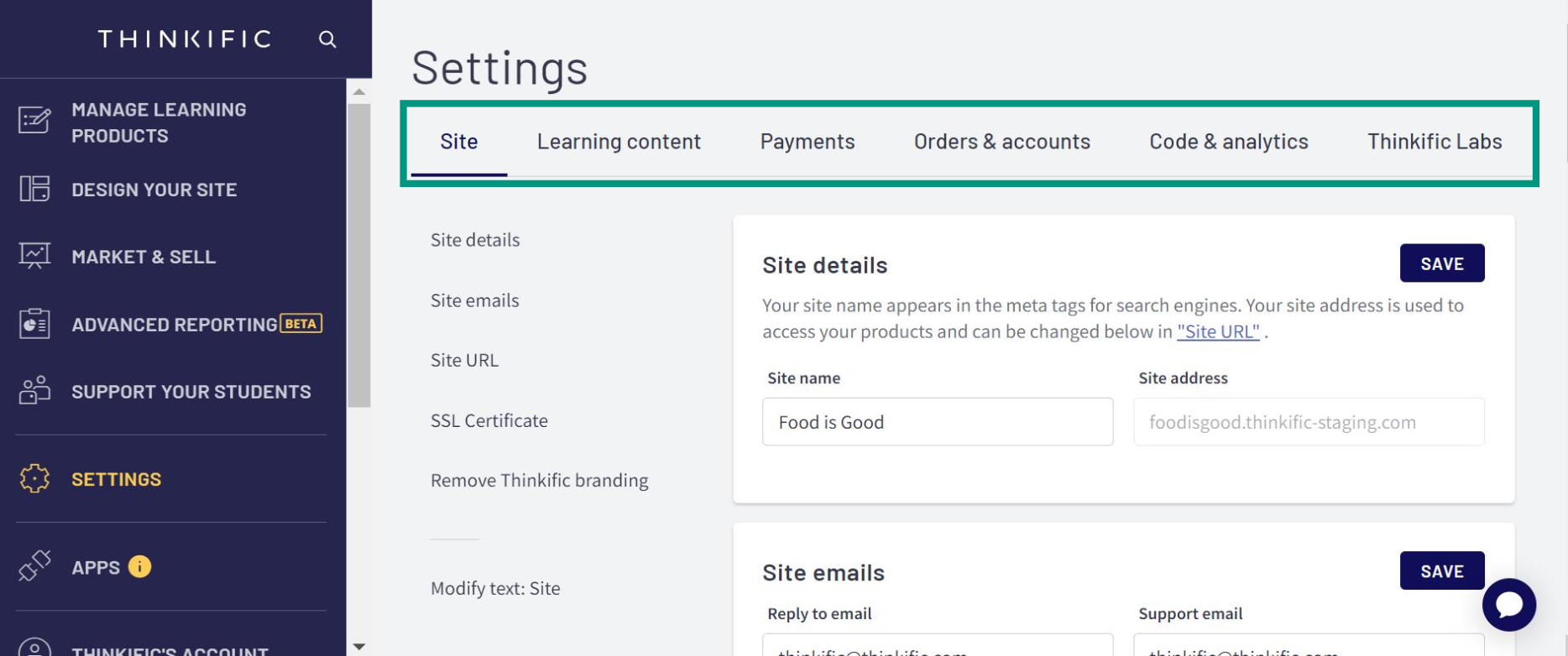The image is a screenshot of a website interface, specifically the dashboard of a site named "Think Thick." In the top left corner, "Think Thick" is prominently displayed beside a magnifying glass icon, likely indicating a search function. Directly below, there is a vertical menu listing the following options: "Manage Learning Products," "Design Your Site," "Market and Sell," "Advance Reporting," "Support Your Students," and "Settings." The "Settings" option is highlighted in yellow, indicating it is the current selection. Below the main menu, there is another section labeled "Apps," marked by a yellow circle with an exclamation mark inside it.

To the right of this vertical menu, there is a content area with a green-tinted rectangle surrounding the submenu items related to "Settings." These submenu items include: "Site," "Learning Content," "Payments," "Return Accounts," "Coded Analytics," and "Thinking Labs."

At the bottom of the screen, additional options are listed on both the left and right sides. On the left, the options include: "Site Details," "Site Emails," "Site URL," "SSL Certificate," "Remove Think Thick Branding," and "Modify Text Site." On the right side, there is a reiterated "Site Details" section. A "Save" button is positioned on the right, with accompanying instructional text: "Your site name appears in the meta tag for each search engine. Your site address is used to access your product and can be changed in Site URL."

The layout and highlighted sections indicate user navigation within the site settings, providing various customization and configuration options for the website.